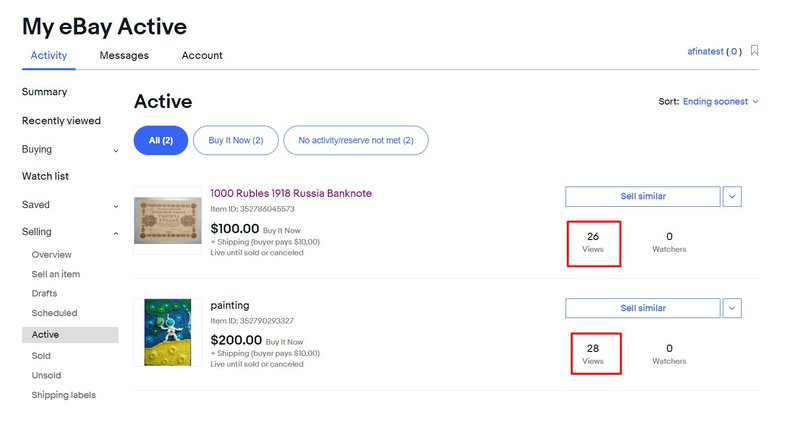This image displays a screenshot of an active eBay user account interface against a white background. 

In the top left corner, the bold text "My eBay Active" is prominently displayed, with 'M' in 'My,' 'B' in 'eBay,' and 'A' in 'Active' capitalized. Directly beneath this, in standard print and underlined in blue, is the word "Activity" with a capital 'A'. 

To the right of "Activity" are three sections in bold black print: "Messages" with a capital 'M,' "Account" with a capital 'A,' and the user’s username "AFINATS," followed by a zero in parentheses. 

The left sidebar lists multiple sections: "Summary," "Recently viewed," "Buying," "Watch list," "Saved," and "Selling." Under the "Selling" section, the options "Overview," "Sell an item," "Draft," "Draft scheduled," and "Active" are displayed, with "Active" in bold print and highlighted by a gray banner. Additional selling options include "Sold," "Unsold," and "Shipping labels."

In the main content area, the word "Active" is again in bold print with a capital 'A.' Below this, a blue banner shows "All (2)," "Buy it now (2)," and "No activity/Reserve not met (2)." Listed are two items: 
1. "1,000 Rubies 1918 Russia Bank Note - $100 - Buy it now"
2. "Painting - $200 - Buy it now"